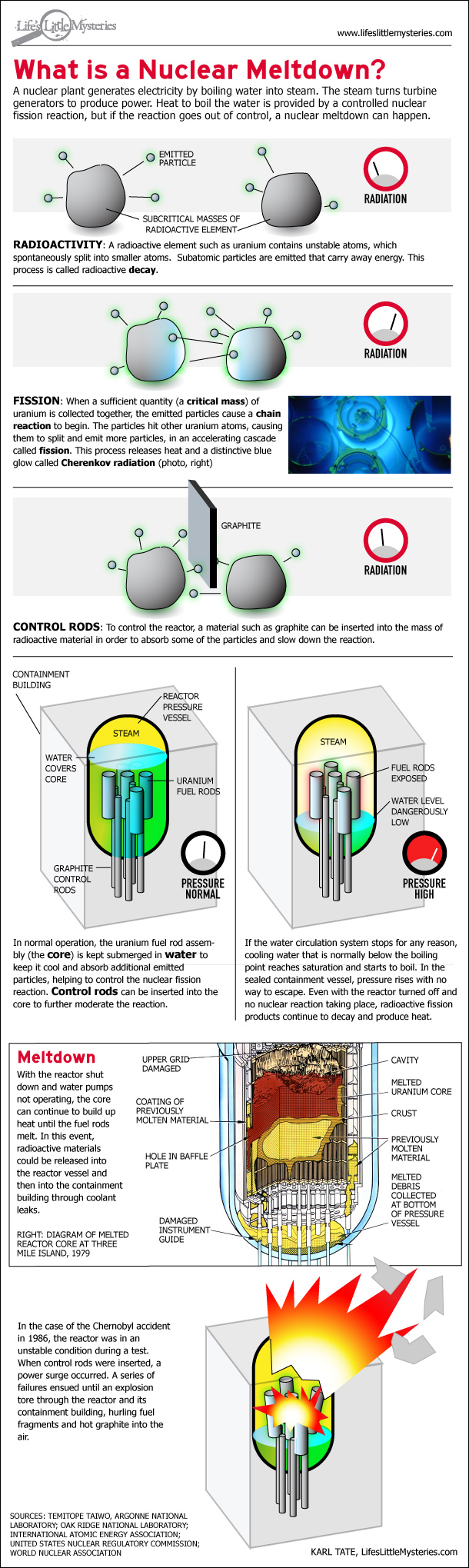This image depicts a detailed vertical diagram likely from a science book or educational wall poster titled in large red letters at the top, "What is a nuclear meltdown?" The poster, much taller than it is wide, methodically explains the stages of a nuclear meltdown through a series of illustrations and accompanying text. The upper sections of the diagram show small gray circles symbolizing radioactivity and an initial step labeled fission. Subsequent sections illustrate control rods and other reactor elements, although the small font makes some details hard to read. Further down, the diagram delves deeper into the process, eventually showing the meltdown phase, depicting a nuclear reactor in the throes of disaster. The final illustration graphically represents an explosion with flames erupting from the reactor. The diagram concludes with a reference to a source, "carltatelifestylemysteries.com," all set against a white background.